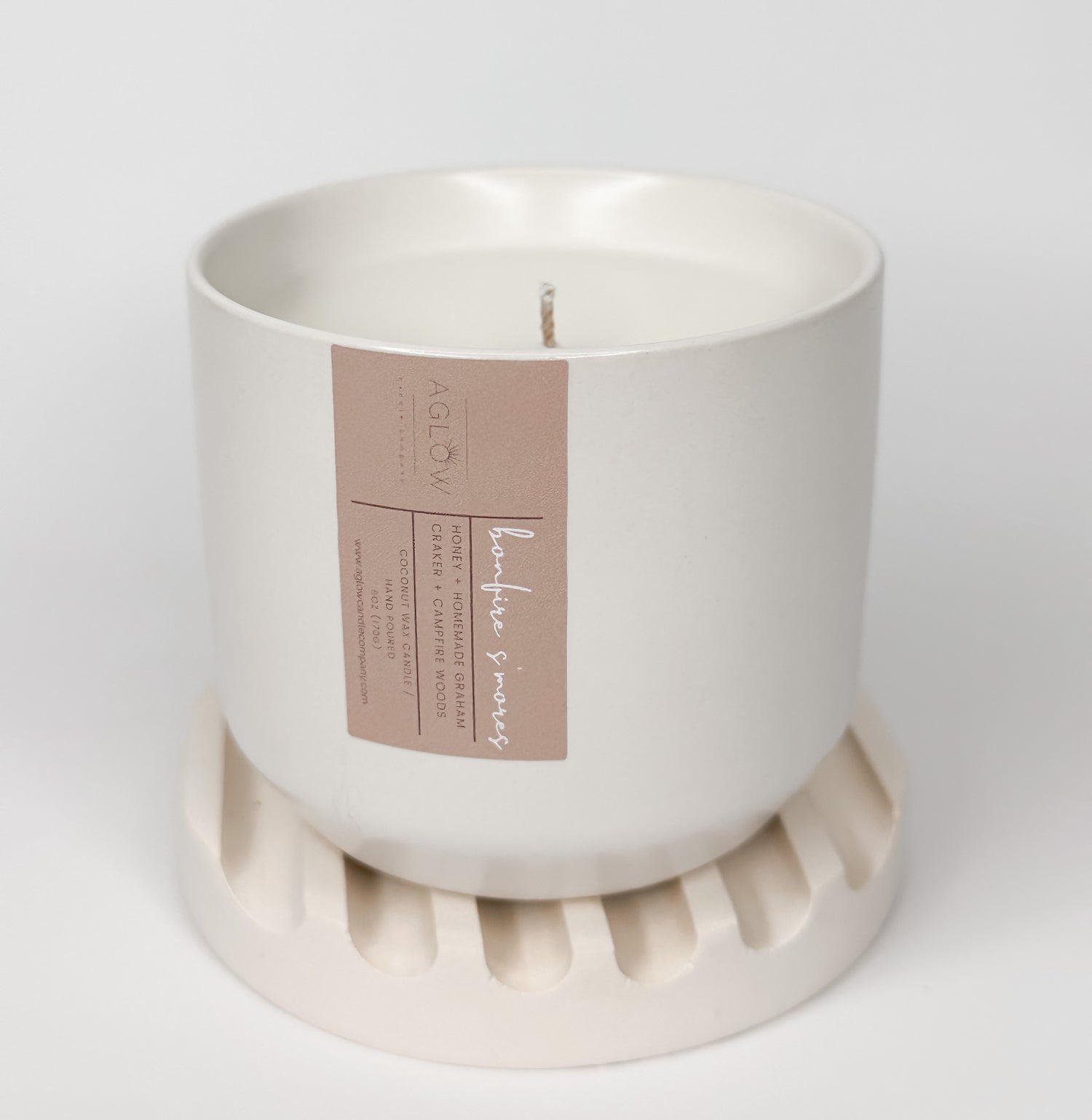This close-up advertising photo features a scented candle in a white glass jar, designed to resemble a coffee cup. The jar holds white coconut wax with a brown wick at its center. The candle, hand-poured by a company named Aglow, exudes a Bonfire S'mores scent, capturing the essence of a campfire with notes of honey, homemade graham cracker, and campfire woods. The label on the jar is a light tan or pinkish hue, displaying the brand name 'Aglow' in black text and the scent name 'Bonfire S'mores' in cursive white text. The container sits atop a cream-colored coaster with indentions for better grip. The entire composition, set against a white background, emphasizes the candle's cozy and inviting aesthetic.